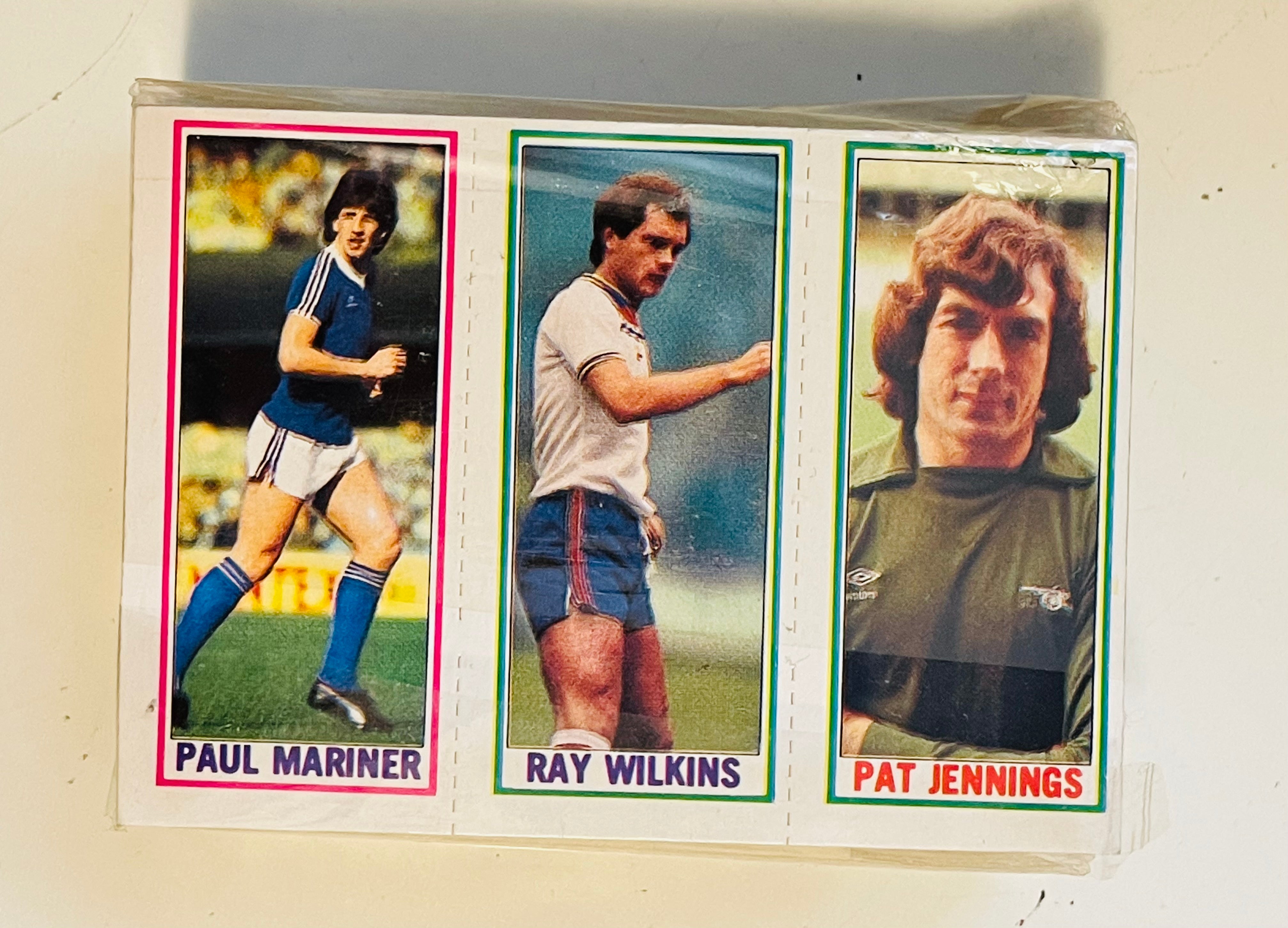The collectible card features three distinct vintage photographs of soccer players, separated by perforated white borders designed for easy tearing. The leftmost photograph is bordered in hot pink and features Paul Mariner, who is running to the right. Mariner wears a blue short-sleeved shirt with white stripes on the sleeves, white shorts with blue stripes, and long blue socks with white stripes. He has fairly long black hair. The central photograph, bordered in dark green, showcases Ray Wilkins in a white short-sleeved shirt and blue shorts with red stripes on the sides. The final photograph, also bordered in dark green, depicts Pat Jennings, identifiable by his long, auburn hair and his dark green long-sleeved shirt. Each player's name is displayed in purple text beneath their respective photographs.